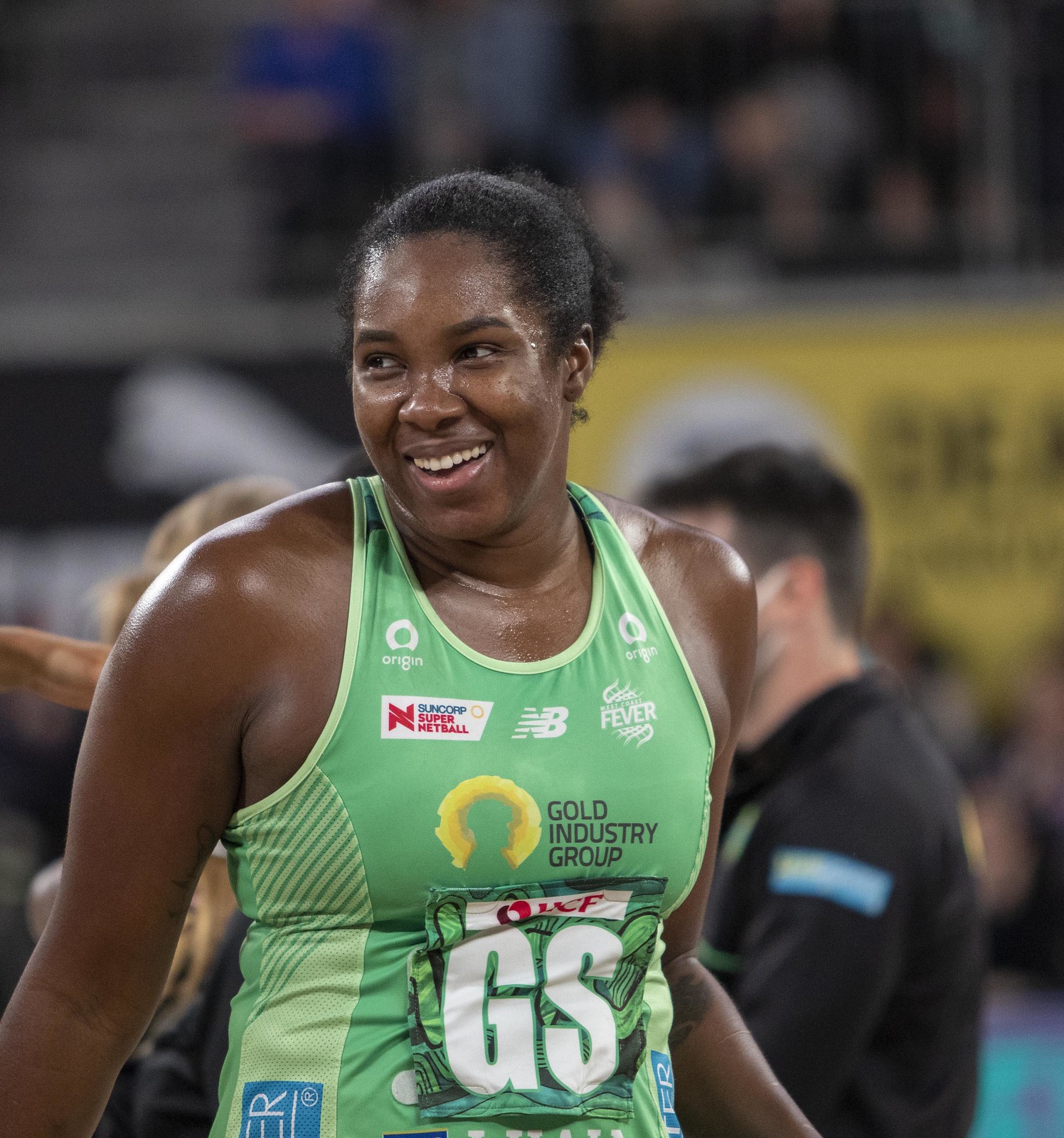The photo captures a young black female athlete, her skin glistening with sweat, standing in a blurred stadium setting that highlights bleachers, indistinct figures, and possibly a yellow sign or banner in the background. She radiates confidence with her hair pulled back into a ponytail and a gleaming white smile as she looks to her left. Wearing a tight green tank top adorned with various sponsor logos such as Origin, Suncorp, Super Netball, New Balance, Fever, and the Gold Industry Group, she exudes the aura of an accomplished sportswoman. The top prominently features big letters 'GS' at the front, with light green stripes running down the sides. The light reflects off her shoulders and face, enhancing her glowing appearance as her arms rest casually by her sides, giving off an impression of motion or preparation in a competitive atmosphere.